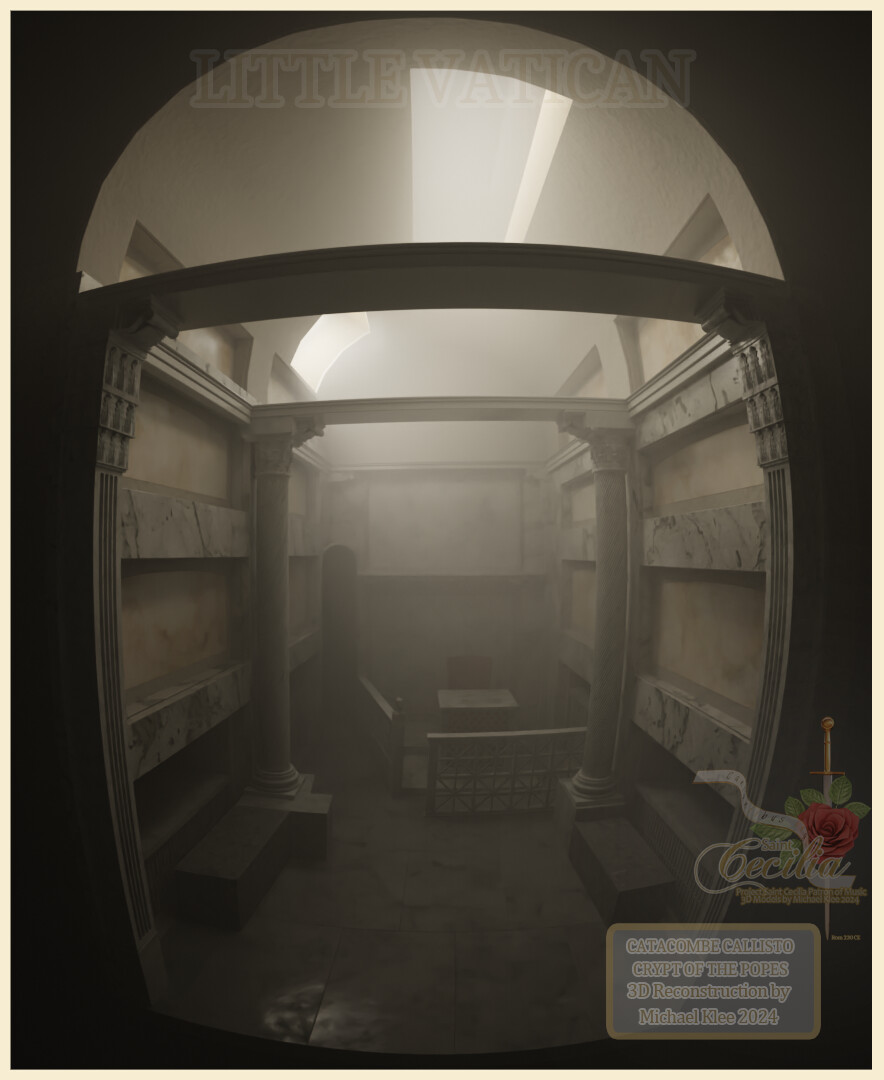The image depicts a detailed, computer-generated reconstruction of an interior setting through a fisheye lens perspective, labeled "Little Vatican" at the top. It appears to be a narrow room with tall walls and marble shelving, possibly resembling a library or study area. The architecture includes an oval-shaped window with a flat bottom, and within the room, there are prominent pillars and benches. A notable feature is a gated section containing a desk. The ceiling is rounded, creating a dome-like effect, and the room is uniformly white. Text within the image reads "Catacomb Callisto Crypt of the Popes 3D reconstruction by Michael Clay, 2024," which is displayed in brown against a light blue background at the bottom corner. The outside details include a rose with the name "Cecilia" inscribed.